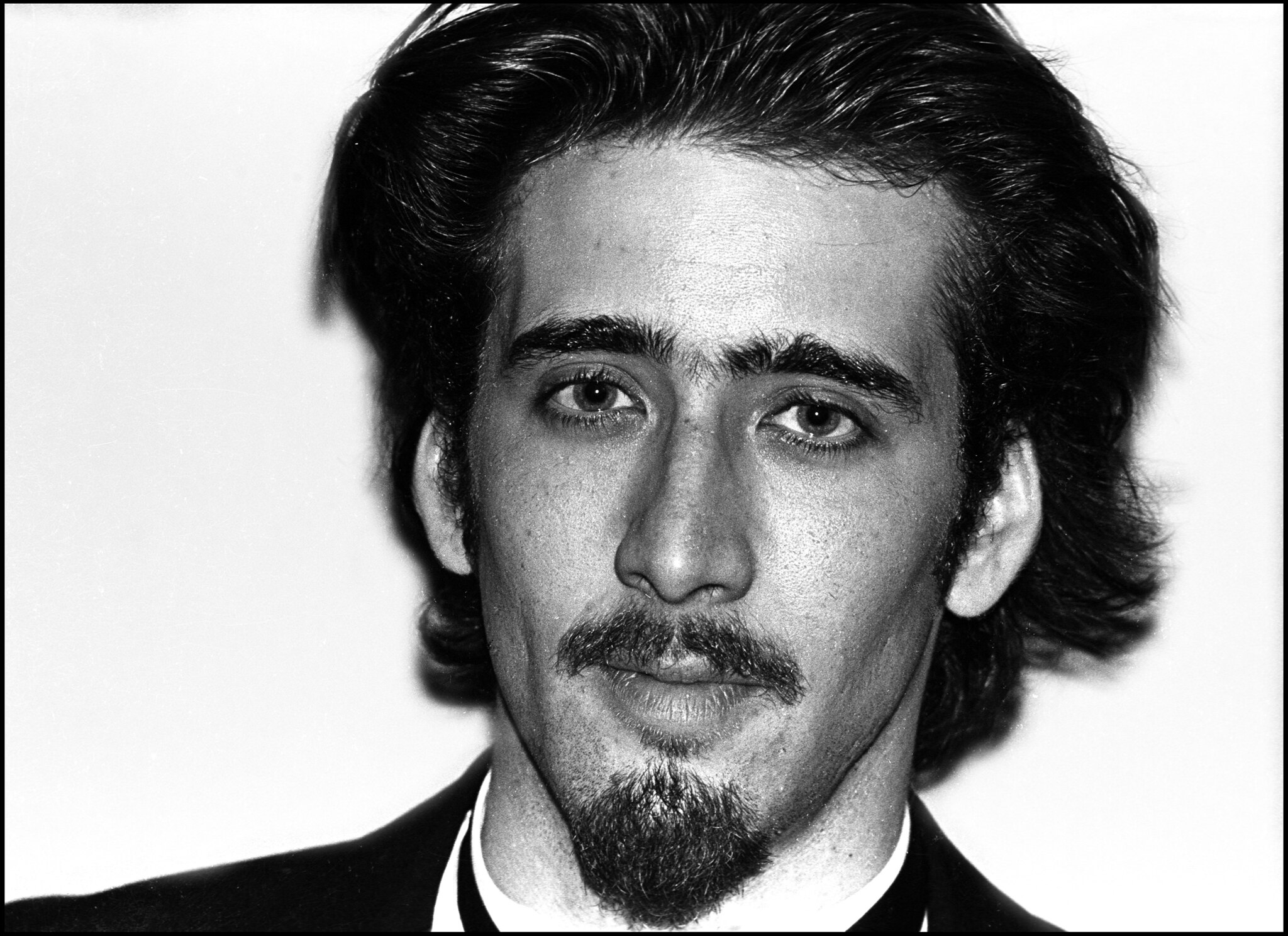This black-and-white close-up photograph from 1984 features a young Nicholas Cage. He is captured from the shoulders up against a plain white background, with the image bordered by a thin solid black line. Cage's thick, dark hair is styled into a mullet, slicked back with gel, adding to the era's distinctive look. His facial features are striking, with thick, bushy eyebrows, prominent long eyelashes, and light brown eyes. He sports a bushy mustache and a thick goatee, covering the top of his lips and accurately defining his rugged appearance. Cage is dressed in a classic black suit, paired with a white shirt and either a white or black tie. He gazes straight at the camera with a neutral expression, perfectly embodying the stoic charm of the era.